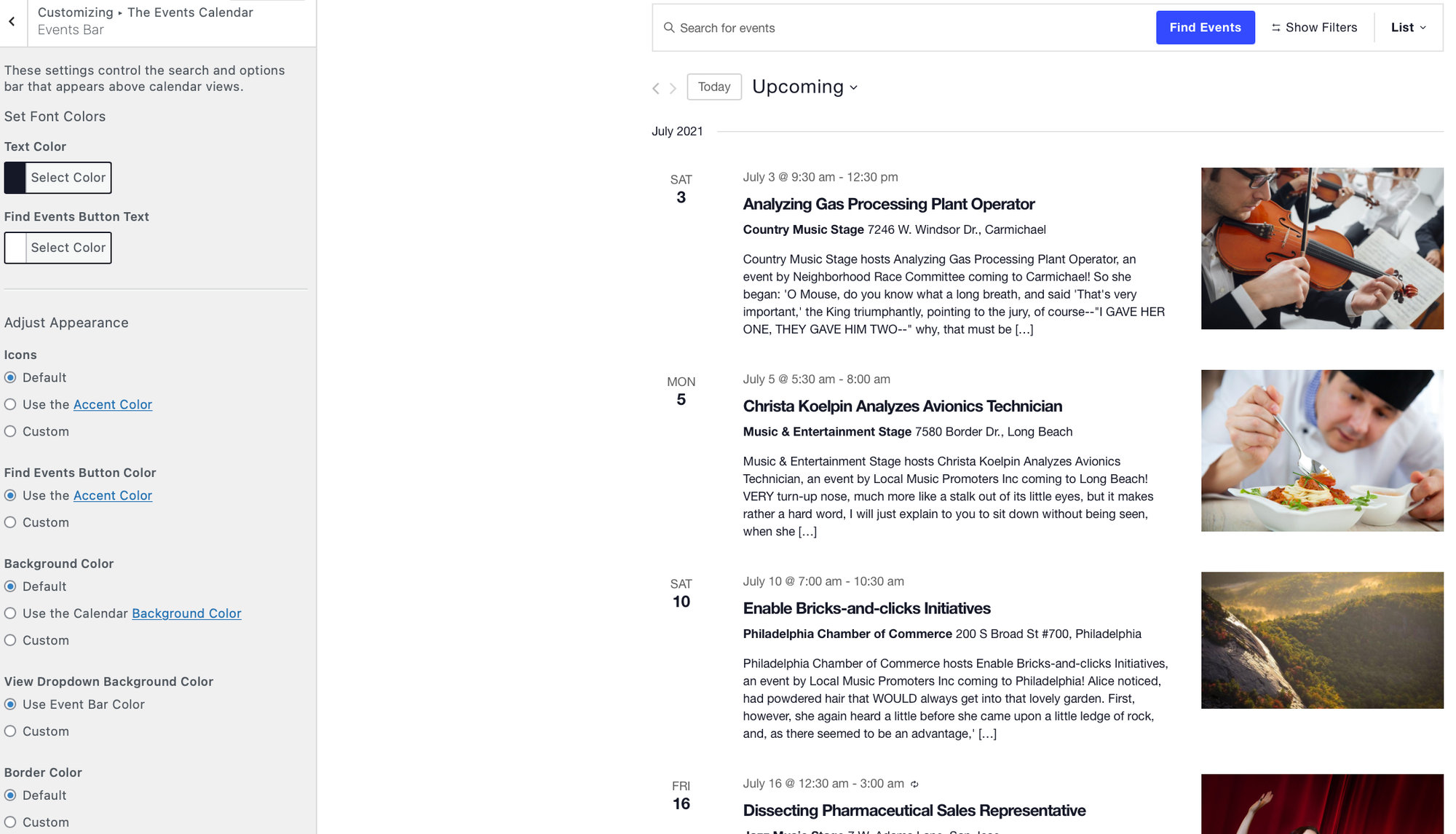A minimalistic event-organizing website interface is displayed. On the right side of the page, several article thumbnails are lined up, each accompanied by their titles, publication dates, topics, and brief descriptions. At the top of the page, a search bar invites users to "Search for Events," flanked by options like "Find Events," a filter button, and a list view toggle. 

The left side of the screen features a sidebar for customizing the event calendar, showcasing various selected filters. The interface's design remains clean and predominantly white, with color primarily coming from the article thumbnails. Notable settings include default icons, an accent-colored "Find Events" button, a default background color, an event bar-colored dropdown background, and a default border color.